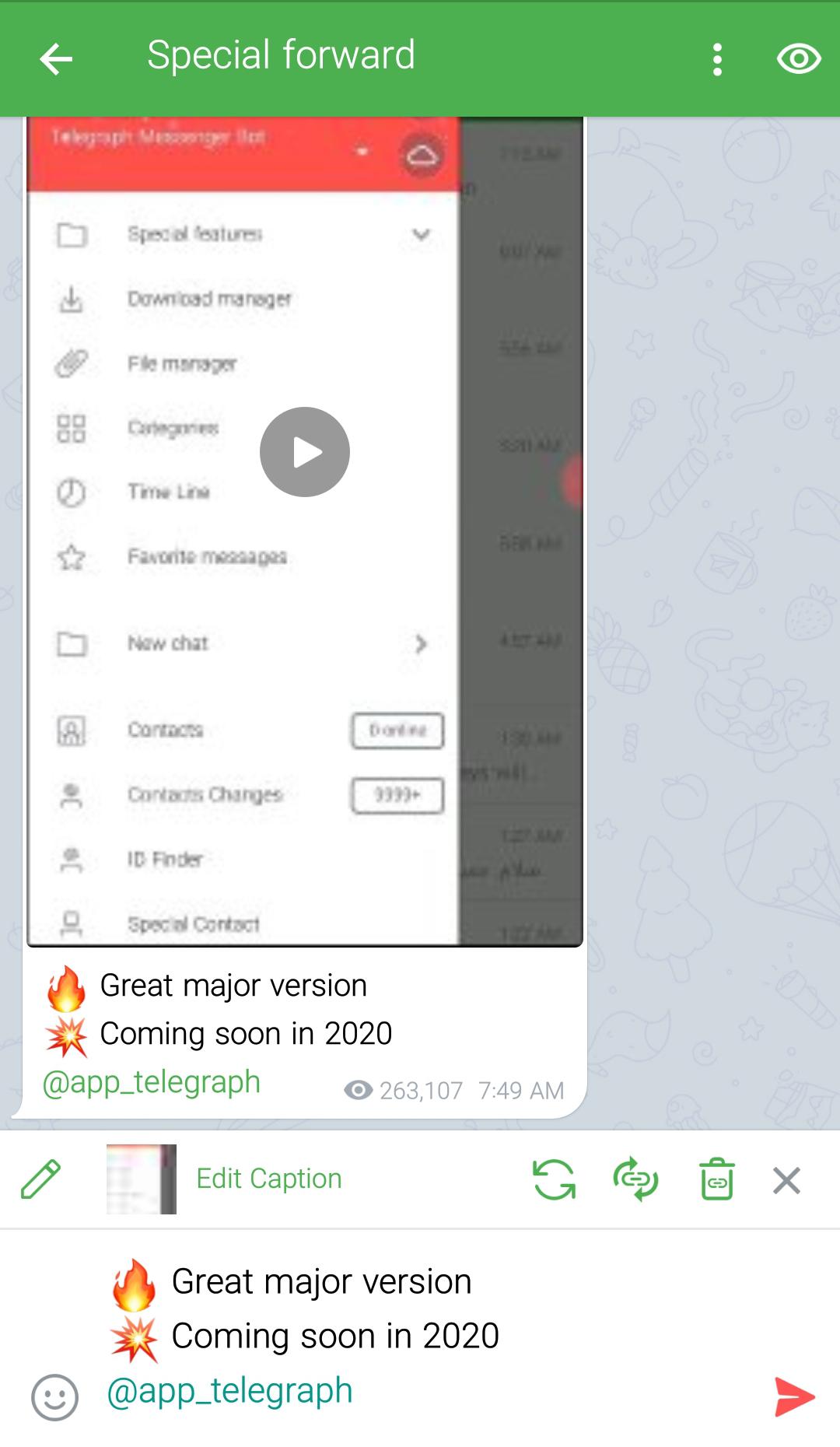The image displays a complex, layered screenshot with multiple interface elements. At the top, there's a green bar featuring a left arrow and the text "Special Forward." Within this, there's an inserted screenshot of a cell phone screen that, in turn, contains another window pop-up. The middle section of the image prominently displays a red banner with the text "Telegram Special Features, Download Manager." To the right of this banner, there's a gray play button icon. Beneath the main elements, there is an illustration of a flame icon next to the text "Great Major Version," followed by a star icon with the text "Coming Soon in 2020 at Telegraph." At the very bottom, there's a section labeled "Edit Caption" that mirrors the text "Great Major Version" and "Coming in 2020 at Telegraph." The arrangement creates a visual effect akin to a picture-in-picture presentation.